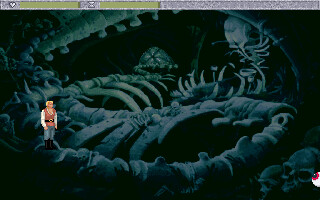This is a color screenshot from an older computer game, showcasing its pixelated graphics. The scene is eerie and unsettling, set in a dark area littered with numerous bones, including several rib cages and two skulls prominently displayed at the bottom right corner. Positioned in the same corner is a macabre detail—a white eyeball with a red iris and a black pupil, adding to the unsettling atmosphere. On the far left stands a character, a man with blonde hair, dressed in a white long-sleeved shirt beneath a red tunic, secured by a black belt with a gold buckle. He wears blue pants and knee-high black boots, and appears to be precariously standing on what seems to be a spine, further amplifying the eerie ambiance of the scene.